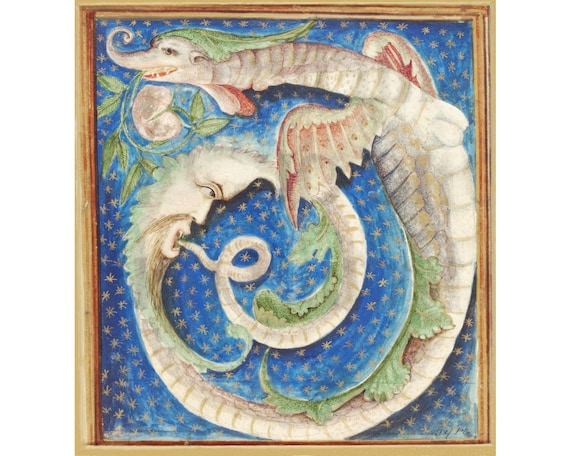This image captures a detailed and whimsical painting of a fantastical European-style dragon set against a deep blue backdrop filled with small, child-like golden stars, evoking a sense of space. The dragon, depicted in pale grayish tones with a hint of green leaves adorning its head and back, features an intricate blend of attributes: its face resembles that of a fish, draped in green leaves, and it carries leaves in its mouth. The dragon's body is long and serpentine, akin to a hybrid between a serpent and a fish. It possesses two large wings and has appendages near its head resembling fins. Uniquely, halfway down its sinuous body, there is a human head emerging, characterized by a long beard, mustache, and fangs, with a somber expression as it swallows the dragon's tail. The painting is framed in a light brown square frame, accentuating its medieval and fairytale-like quality.